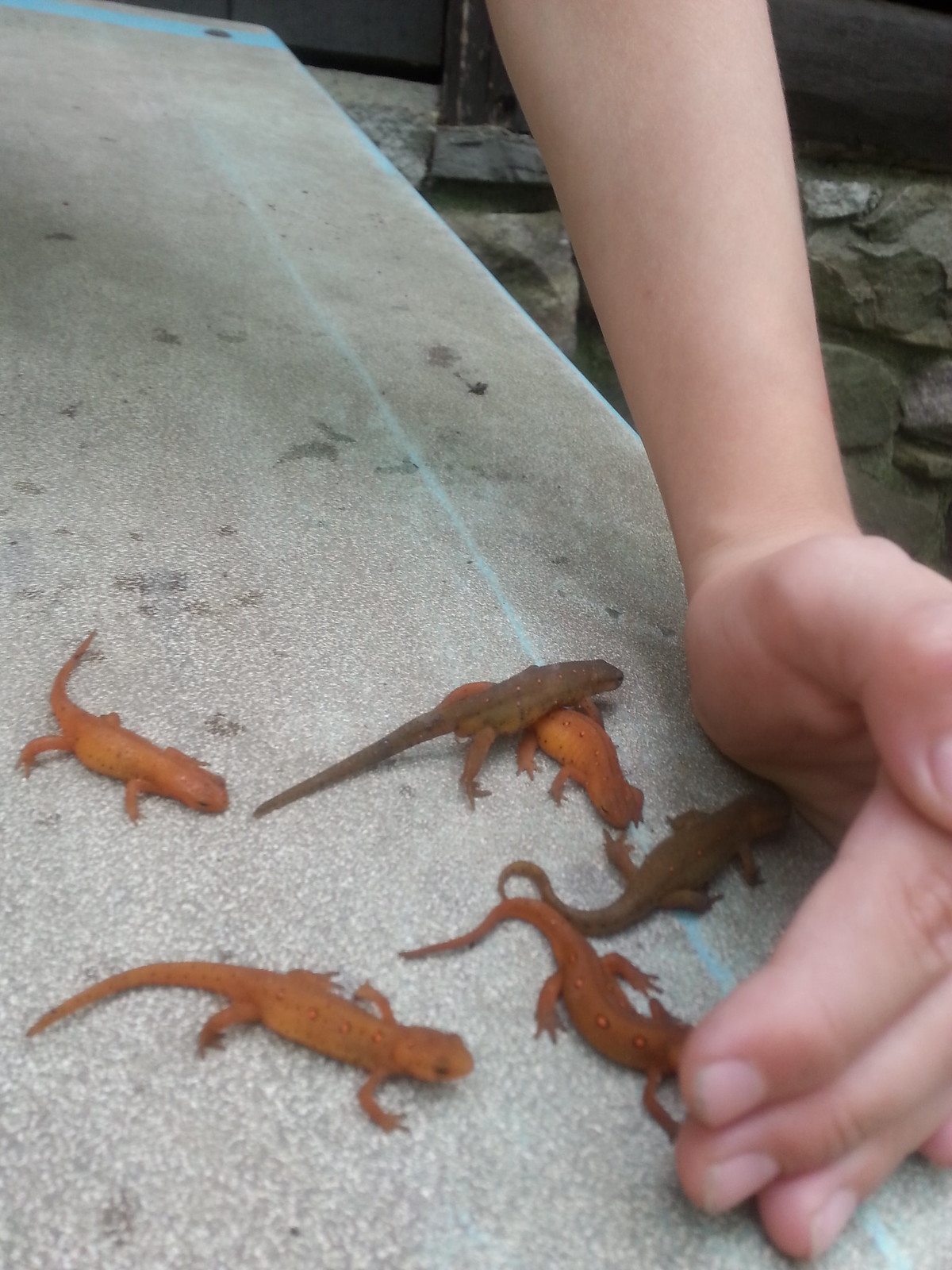The image captures a small group of six lizards crawling on a stone structure that appears to be a wall constructed from concreted rocks. The lizards are of varying colors, with three at the front being an orangish color with darker, reddish spots dotted with tiny white specks. Another one has a darker brown shade near a person's thumb. There is one lizard climbing over another in the second row, heading towards the person's hand, while another lizard slithers towards the front bottom of the picture. The last lizard is positioned in the middle-left area of the image. The person's hand, seemingly cupped to prevent the lizards from escaping, extends down from the top right, revealing only the arm from the elbow down. A faint blue streak runs horizontally across the upper left corner and along the middle edge of the picture, adding a subtle background detail. The setting looks like it could be part of a bridge, sidewalk, or near a water body such as a pond or creek.